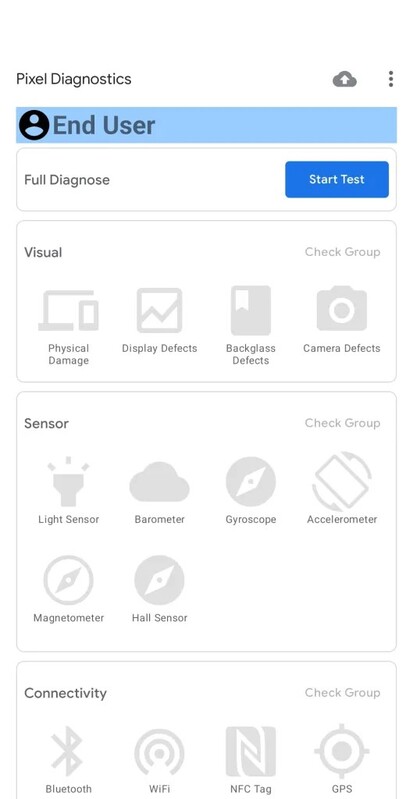The image presents a detailed interface for "Pixel Diagnostics" on a white background. At the top left, the text "Pixel Diagnostics" is displayed in black. On the top right, there's a gray cloud icon symbolizing user options, accompanied by three vertical dots.

The main interface is embedded in a bluish rectangle. Within this rectangle, there is an outlined icon of a person in black. Below the icon, "UserIn" is written in dark blue. To the right, there is a button labeled "View Diagnostics."

On the right side, a prominent blue square with white text reads "Start Test." Adjacent to it, another square in white shows the word "Visual." Below this, several diagnostics options are listed in lighter font:
- Physical Damage
- Displayed Defects
- Glass Defects
- Camera Defects

Each of these options is accompanied by corresponding icons illustrating the respective issues.

The next section, titled "Sensor," is displayed in black text. The listed sensor diagnostics include:
- Light Sensor (represented by a flashlight icon)
- Barometer (illustrated with a cloud)
- Gyroscope (depicted as a compass)
- Accelerometer (shown with a phone tilting left and right)
- Magnetometer (an outlined compass icon)
- Hall Sensor (another compass icon)

Under the section labeled "Connectivity," the diagnostics include:
- Bluetooth (Bluetooth symbol)
- Wi-Fi (Wi-Fi symbol)
- NFC Tag (outlined "N" symbol)
- GPS (represented by a compass with North, South, East, and West directions, though not explicitly labeled, with a central circle)

This image effectively concludes the information available for this diagnostic interface, without any additional content beyond what has been described.